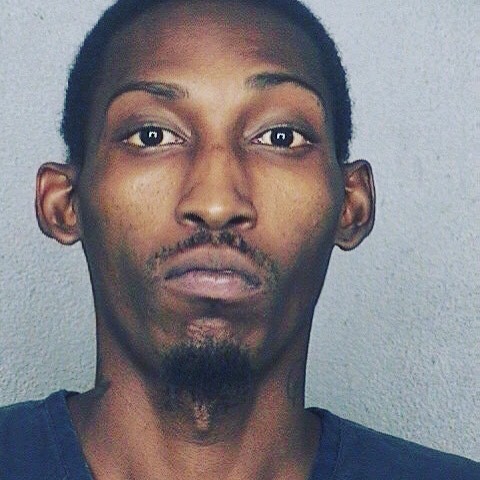This image is a close-up photograph of an African-American man with dark skin. He has short, closely cropped, curly black hair and dark brown eyes with matching brown eyebrows. His facial hair includes a small, thin black mustache and a small beard just on his chin. His ears stick out slightly. He appears very serious and is not smiling. The man is wearing a navy blue shirt, and the background is a light, mostly gray wall.

Distinctive features include tattoos on his neck, one visible on the left side which appears as a line within a circle, and possibly another on the right side, although it could also be shadowing. His Adam's apple is noticeable and appears slightly paler compared to the rest of his skin. His cheekbones are pronounced. The overall impression is of a somber, composed individual.